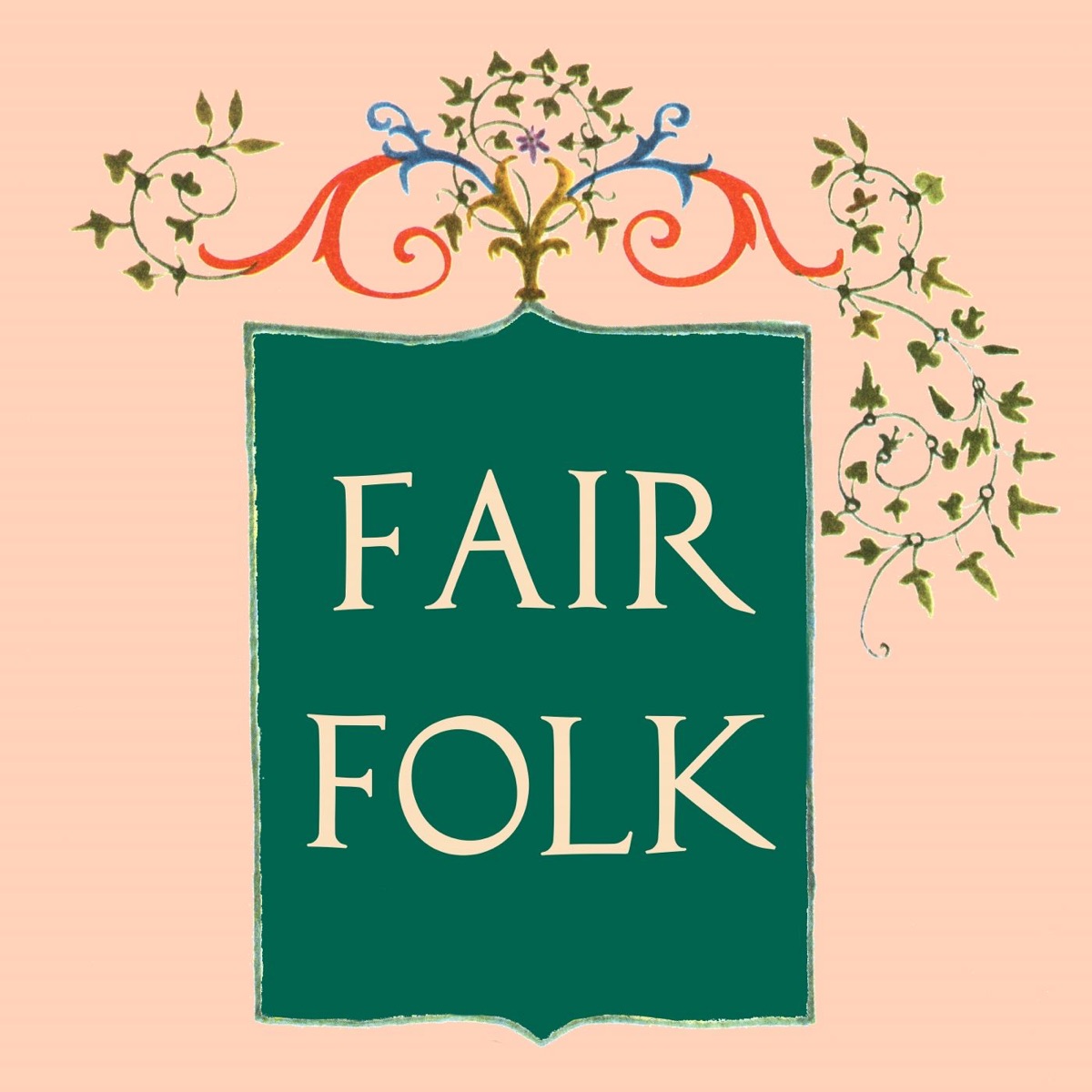This is an artistic illustration featuring a central sign that states "Fair Folk" in white, all-caps text. The text is set against a blue teal background, shaped slightly like an open book, with a faint light trim that transitions to a pastel peach-pink backdrop. At the top of the blue teal shape are swirling vines that evoke an intricate, stylized fleur-de-lis design. These vines boast a vibrant palette with green, red, blue, and gold hues, and they end with trident-shaped leaves reminiscent of English ivy. The central vine also sports a singular purple flower. This detailed composition melds the serene tones of the pastel background with the vivid, dynamic scrolls and foliage, creating a visually captivating and whimsical scene.